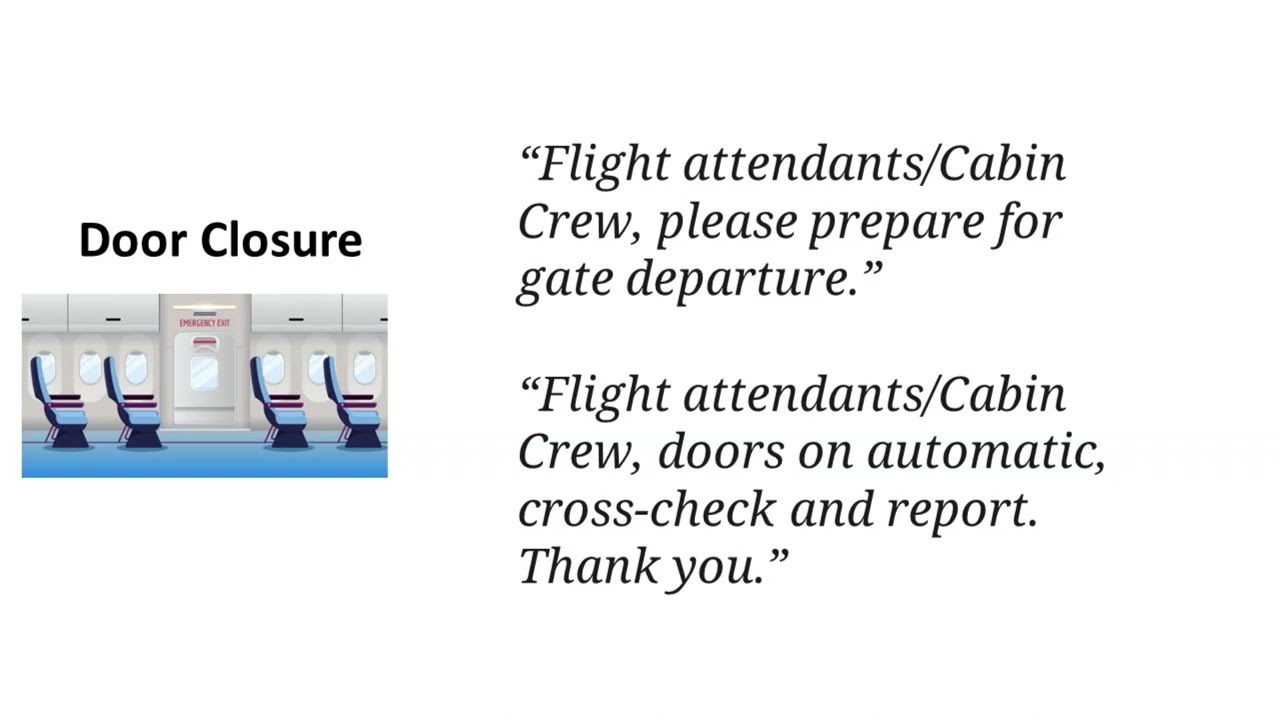The image depicts an informational brochure page with a white background. On the left side, there is a small, horizontal digital image illustrating the interior of an airplane. This image shows rows of seats with blue fabric, blue carpet, and small oval windows. A rectangular vertical emergency exit door is visible between the seats. Above this image, the heading reads "Door Closure." To the right of the airplane illustration, two sets of instructions are written in black text encased in quotation marks: "Flight attendants/cabin crew, please prepare for gate departure." Below this, the second instruction reads, "Flight attendants/cabin crew, doors on automatic, cross check and report. Thank you."